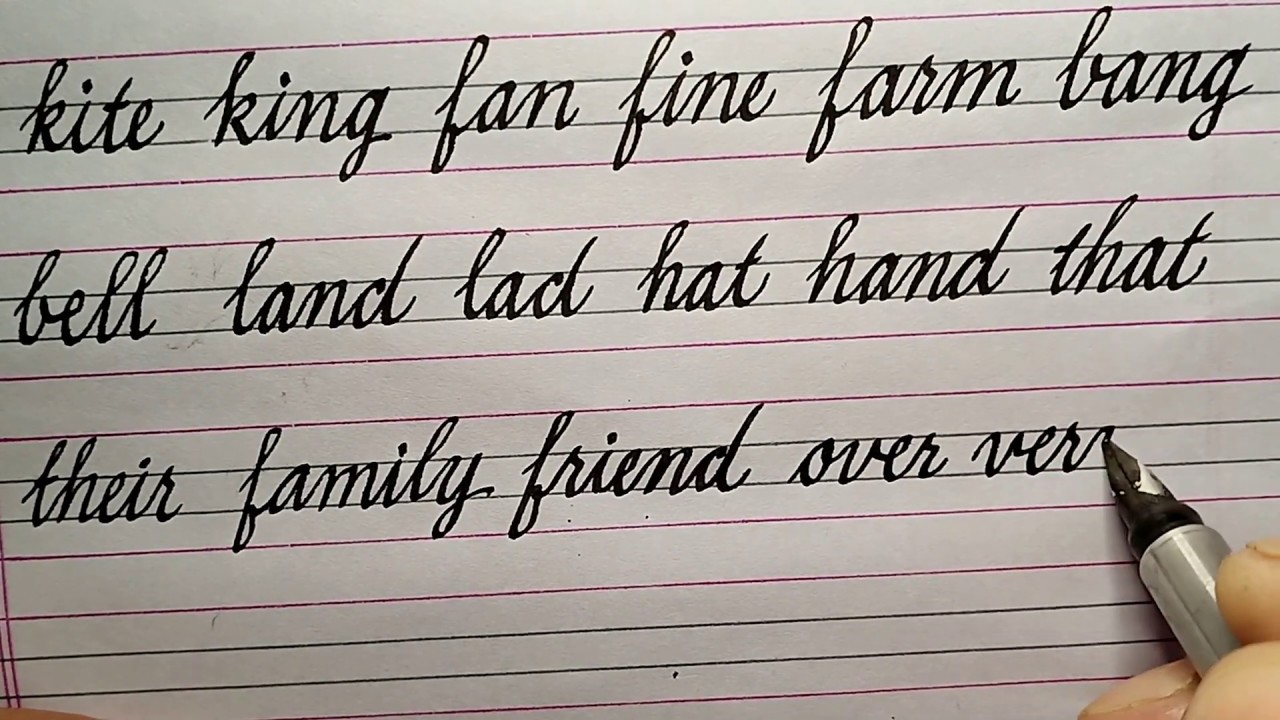In the image, someone is practicing their cursive writing on a lined piece of paper that appears to have a slight pinkish or lavender tint. The paper features traditional pink and black guidelines. The writing is in black ink, produced by an ink pen with a split tip. Visible in the bottom right corner of the image are a couple of fingers holding the pen as the person starts to write the word "very." The text already written on the paper includes the following words: kite, king, fan, fine, farm, bang, bell, land, lad, hat, hand, that, their, family, friend, and over. The cursive writing takes up approximately 70% of the page, and though the photo itself has a darker tone, it showcases the horizontal, neat cursive text against the lined background.